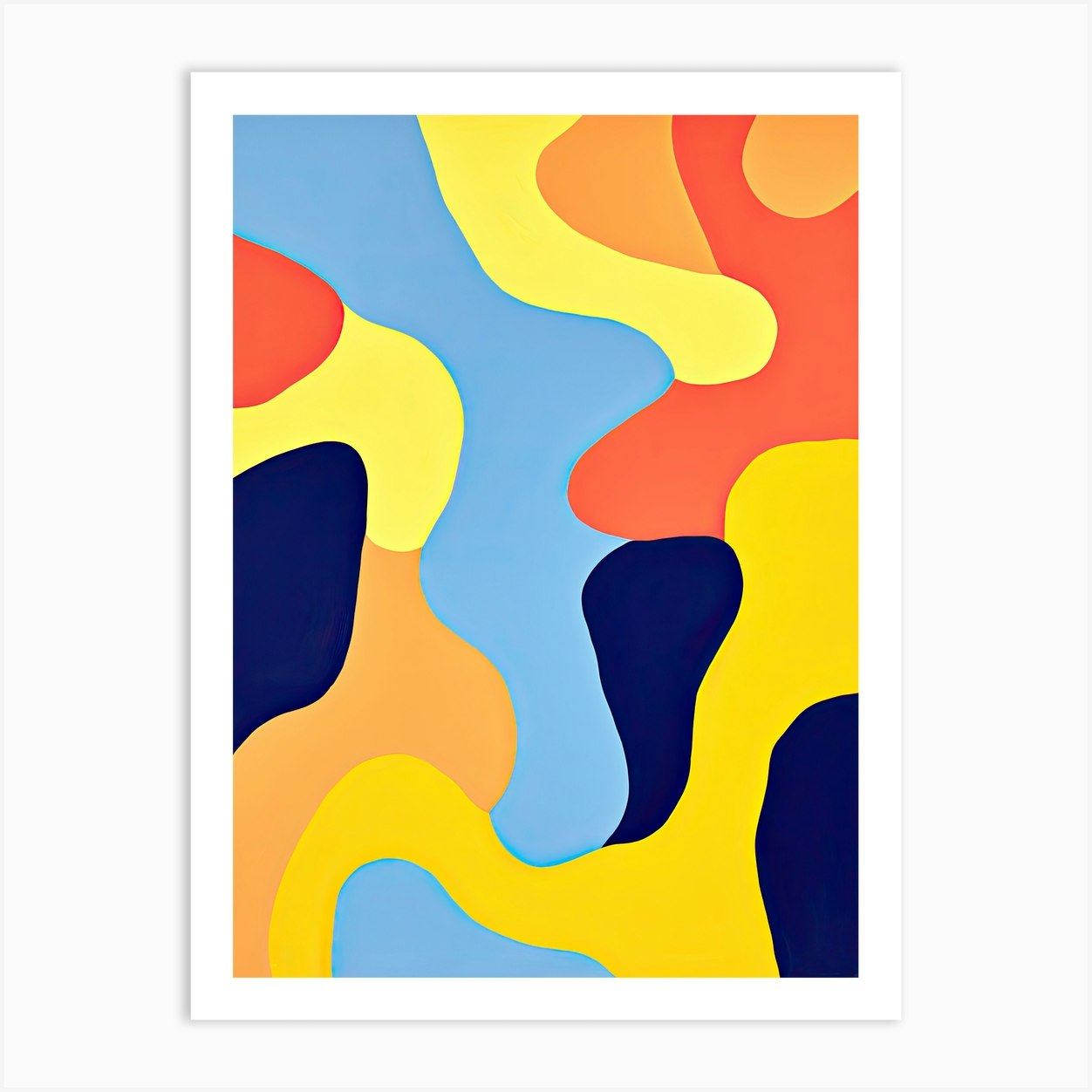The image presents an abstract digital artwork or painting mounted on a white wall, characterized by its simplistic yet fluid design. The central white canvas is adorned with a series of wavy, squiggly patterns reminiscent of the organic forms found in lava lamps or oil spills. These patterns encompass a vibrant spectrum of colors, including shades of yellow, reddish-orange, blue, navy blue, and black. The colors appear to blend and bleed into each other in a seemingly random yet harmonious manner, suggesting an impromptu or spontaneous artistic approach. The entire piece is encased in a solid white frame, which contrasts and highlights the vividness of the colors within. Despite the differing opinions on its execution, the artwork stands as a minimalist yet striking composition of fluid, colorful waves and squiggles against an immaculate backdrop.